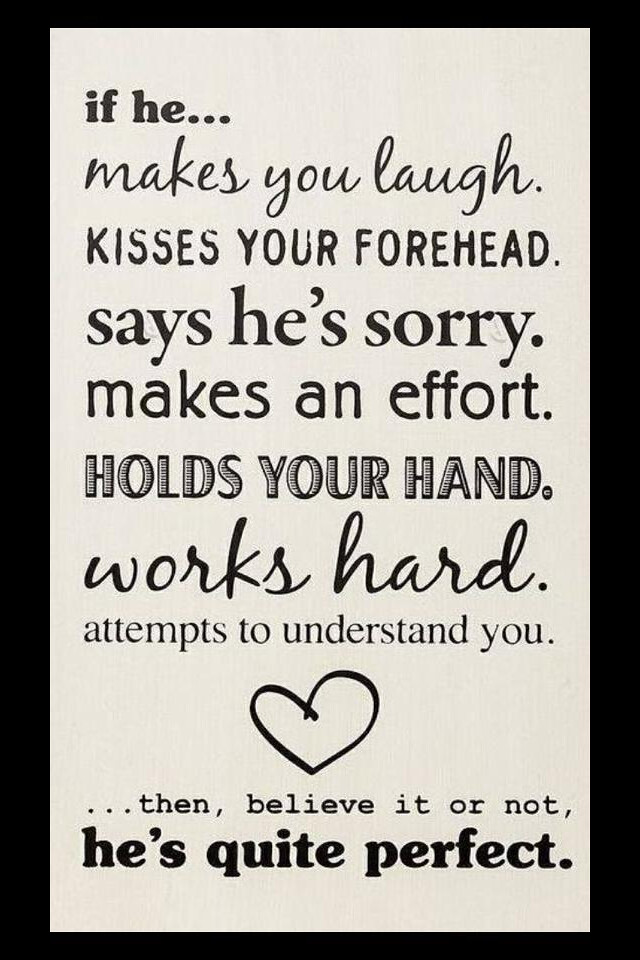The image is an illustration of a motivational quote designed to be a decorative wall hanging. It features a muted white, slightly beige background with black text arranged in a visually appealing format. Each line of the quote is in a different font, giving it a dynamic and varied look. The quote reads:
 
"If he
makes you laugh,
kisses your forehead,
says he's sorry,
makes an effort,
holds your hand,
works hard,
attempts to understand you (stylized heart symbol),
then believe it or not,
he’s quite perfect."

The final line, "he's quite perfect," is emphasized with a big, bold font. This piece conveys a sense of wisdom and encouragement, making it suitable for display in a home setting, much like the popular "Live, Laugh, Love" décor.